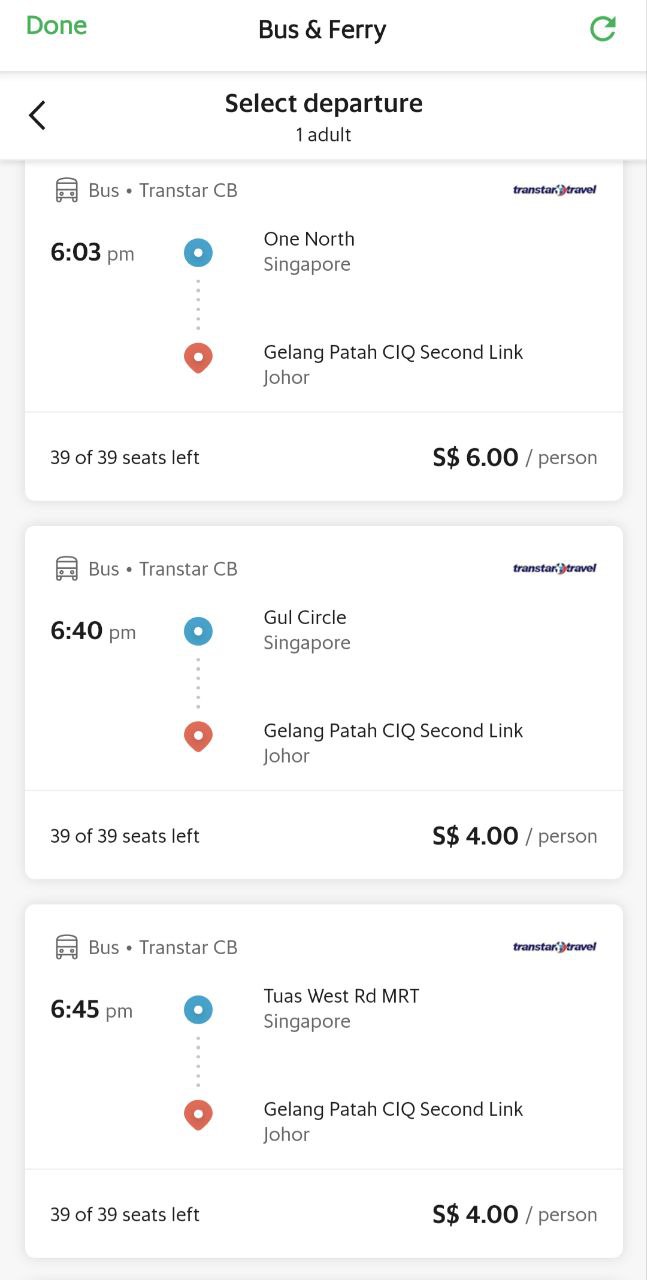The image depicts a booking page for bus and ferry transportation. At the top, the header reads "Bus and Ferry." In the upper left corner, there's an option labeled "Done." The main section lists various bus transfer options with their details.

1. The first bus transfer is listed as:
   - Time: 6:03 PM (CB603pm)
   - Route: One North Singapore to Jalan Pata CIQ Second Link.
   - Price: $6 per person.
   - Availability: 39 out of 39 seats left.

2. The second bus transfer is listed as:
   - Time: 6:40 PM.
   - Route: Jalan Pata CIQ Second Link.
   - Price: $4 per person.
   - Availability: 39 out of 39 seats left.

3. The third bus transfer also departs at 6:40 PM, with the following details:
   - Route: Charles West Road, MRC Singapore to Jalan Pata CIQ Second Link.
   - Price: $4 per person.
   - Availability: 39 out of 39 seats left.

Overall, this booking page allows users to select their departure, view the available options, and complete their reservations for bus and ferry services.